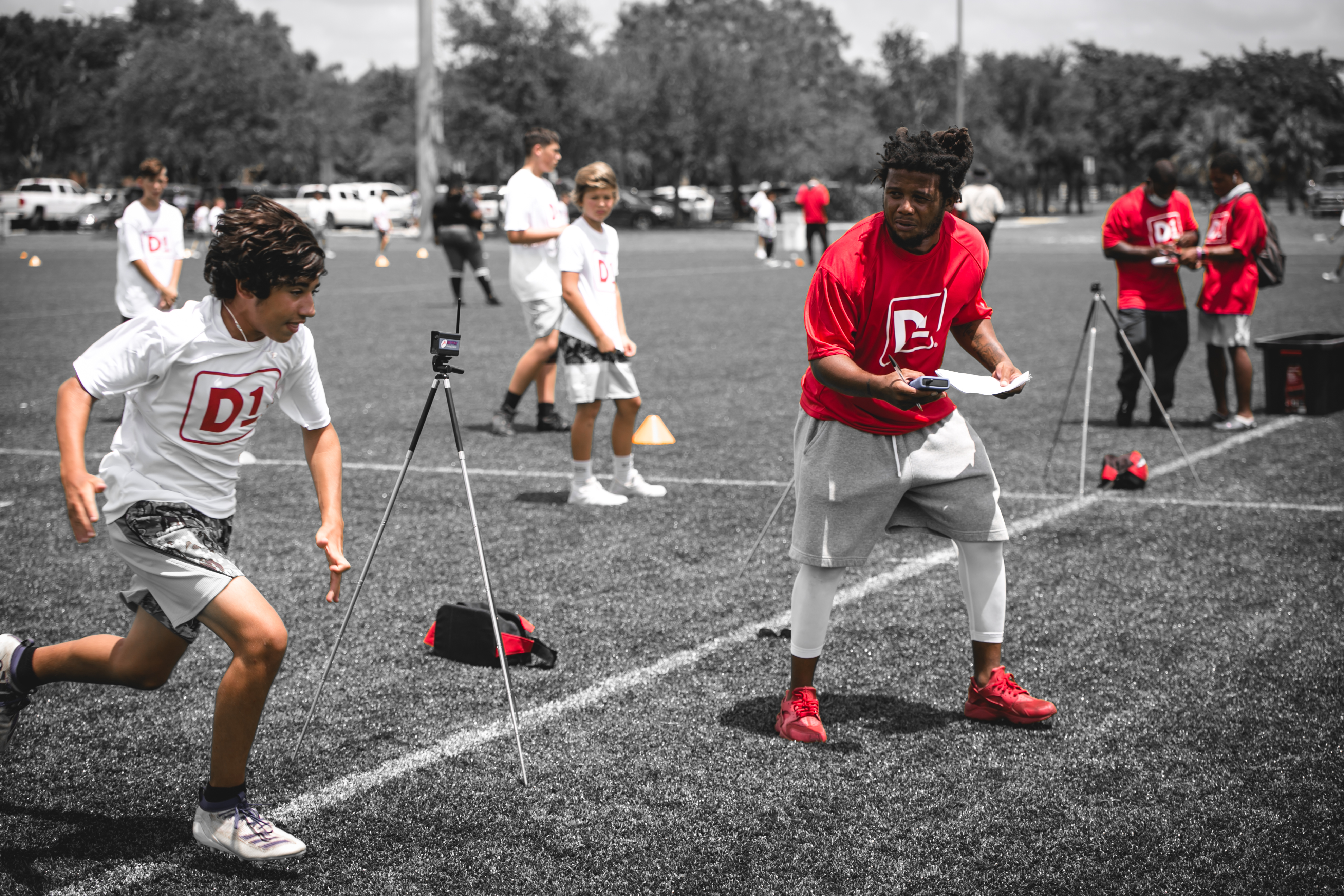This outdoor scene captures a vividly edited image of what appears to be a soccer tryout or practice session. The setting occurs on a field where all participants and coaches are displayed in vibrant colors, contrasting starkly with the monochrome black-and-white background of grass, trees, and sky—a likely result of photo editing to make the people pop. There are several young men, dressed uniformly in white t-shirts featuring the D1 logo within a red-bordered rectangle and gray shorts, scattered across the field. Among them, only one player's logo is fully visible, but it is clear that all shirts bear the same design. The coaches, distinguished by their red shirts with a similar D1 logo, watch over the players. One coach, dressed in red with gray shorts and red shoes, appears to be timing a player who is actively running, perhaps using a stopwatch. Multiple tripods, potentially holding cameras or timing devices, are strategically placed around the field. The racial diversity among the group is identifiable, with coaches of black skin, and players of white and brown skin tones. The scene is pulsating with the energy of sportsmanship, caught in a moment of instructional focus amidst the striking color contrast.